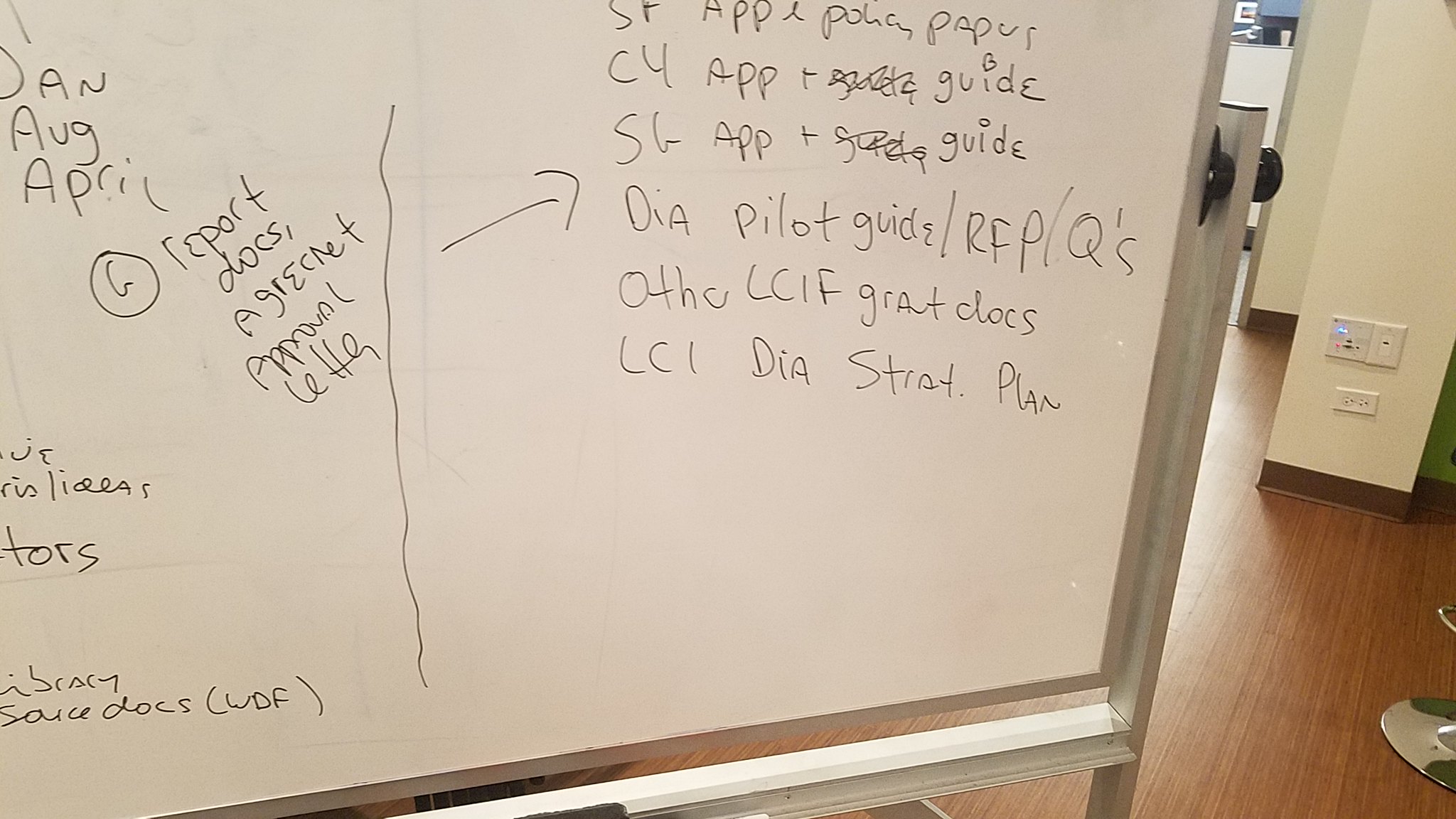This is a horizontal rectangular photograph capturing a large whiteboard set against a white wall within a spacious room with a brown hardwood floor. The whiteboard, framed with silver edges, is prominently positioned, partially obstructing the view of the room, with only a corner of the back wall and an electrical outlet visible on the right. In the lower right corner of the image, a foot is noticeably peeking into the frame.

The whiteboard itself is covered with extensive black marker writing, which appears to detail various study notes or information potentially related to pilot training. However, the majority of the text is either illegible or difficult to decipher. Clearly visible on the left side of the board are terms such as "Jan, Aug, April," followed by a circle marked with a "C," "report docs," and "green approval letter." Continuing downward, the board lists "AppPAPIS," "AppGuide" repeated twice, "DyaPilotGuide," "RFPQs," "LCIF grad docs," and "LCIDIA stray plan." The cluttered writing and numerous arrows connecting different points give the impression of a complex, in-depth lesson or briefing session.